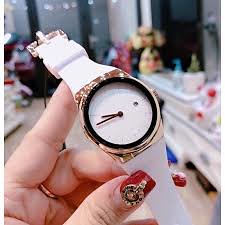This indoor color photograph, taken from above, captures a detailed close-up of a woman's left hand holding a wristwatch. The wristwatch features a round white face encircled by a black ring and is devoid of any numerals; instead, it has black dashes to indicate the hours and black hour and minute hands showing the time as approximately 14 minutes to 10. The watch's bezel and buckle are gold-toned, and the strap is white, possibly made of leather or a heavy plastic. The woman’s ornate red fingernails feature intricate gold patterns, with her thumb positioned just below the watch face and her middle finger and pinky holding the bottom of the band, while her pointer finger supports the upper part. The background of the image appears to be a blurry store setting, possibly showing a countertop and windows. Additionally, the woman is wearing a gold ring on her pointer finger.